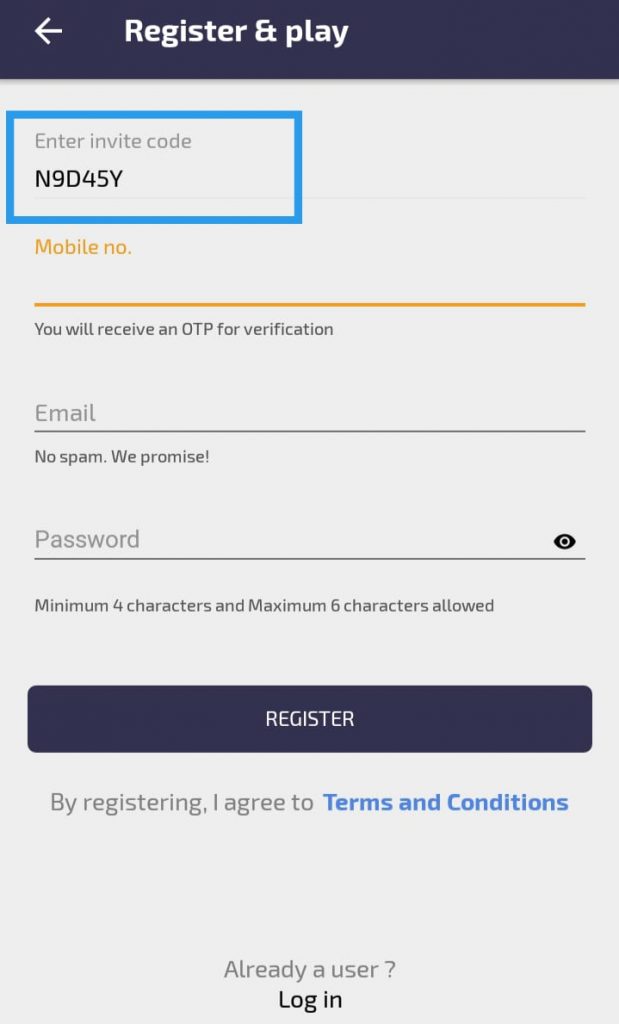The image is a screenshot of a "Register & Play" page with user input fields and registration information. 

The background is a light shade of gray, and a navy blue banner spans the top of the page. Within this banner, on the left side, there is a white left-facing arrow icon. To the right of the arrow, the text "Register & Play" is displayed, with "Register" and "Play" separated by an ampersand symbol.

Below the banner, a blue rectangular box highlights a section where users can enter an invite code. This section contains the placeholder text "Enter Invite Code" in light gray, and beneath it, the code "N9D45Y" is shown. Users can enter their invite code on a thin gray line beneath this text.

Following the invite code section is an input area for a mobile phone number. The label "Mobile No." is written in orange text, accompanied by an orange horizontal line where the mobile number can be entered. Currently, no number is entered in this field. Underneath, a fine print note informs users that they will receive a One-Time Password (OTP) for verification.

The next section is for entering an email address. It includes the placeholder text "Email" in light gray, sitting above a gray dividing line. Directly below this line, there is a promise of "No spam. We promise!"

Below the email address input is a section for creating a password. It too has the placeholder text "Password" in light gray, above a gray dividing line. On the rightmost edge of this section, a black eye symbol serves as a privacy icon, likely indicating that users can toggle the visibility of their password. A note beneath this section specifies that the password must be between 4 and 6 characters.

Near the bottom of the page, a navy blue "Register" button spans almost the entire width of the page. Below the button, a disclaimer reads, "By registering, I agree to Terms and Conditions," with "Terms and Conditions" highlighted in light blue.

At the very bottom center, there is a small text prompt for existing users: "Already a user? Login," with the word "Login" in black text.